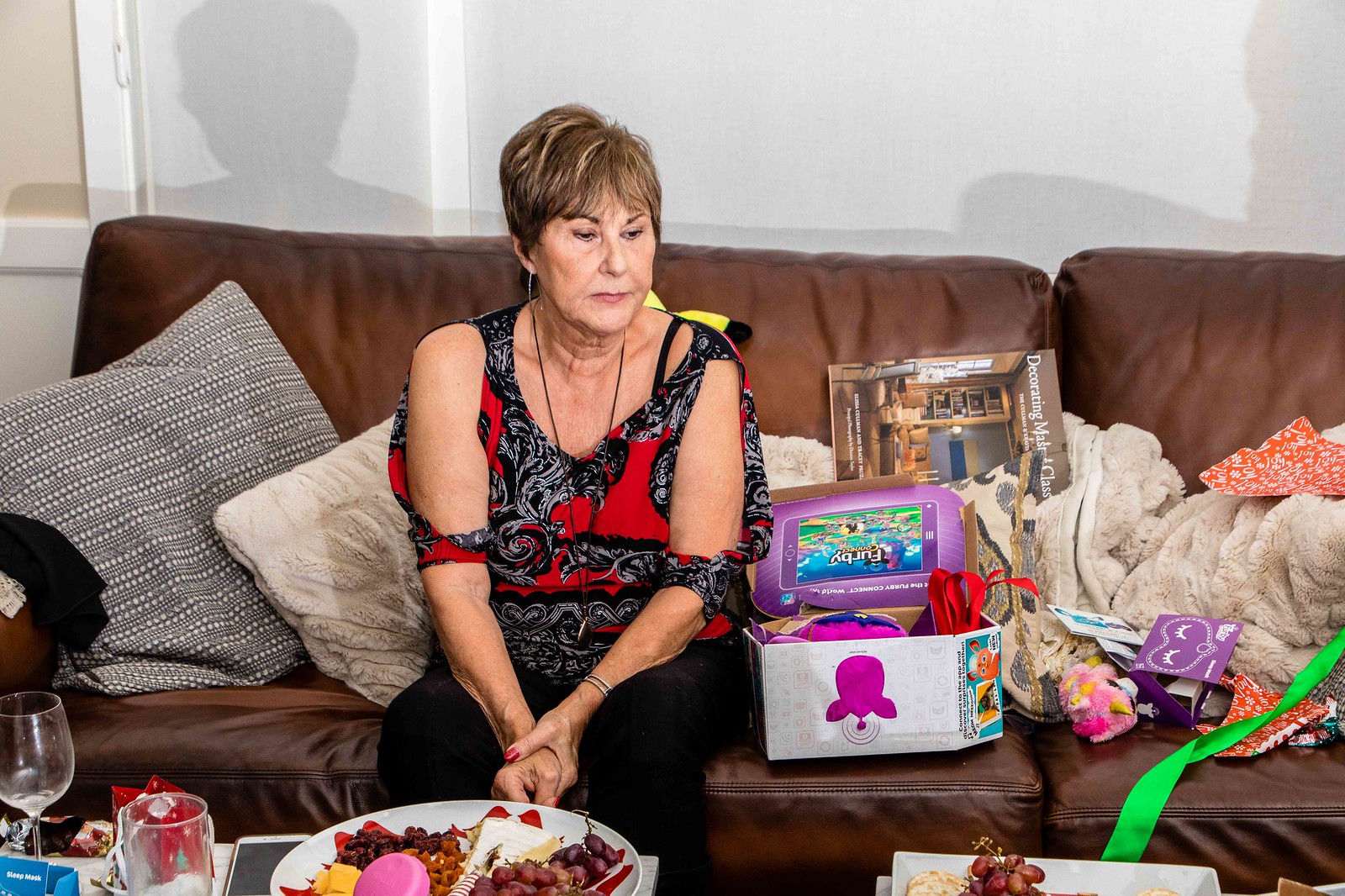The image depicts a white woman with short brown hair seated on a brown leather couch, slightly left of center. She is dressed in black pants and a red cold-shoulder top adorned with black and white patterns. Her stern or possibly sad expression contrasts with the vibrant red nail polish on her fingers. Behind her, two pillows—one gray and one white—and a tan blanket are visible, complementing the white wall in the background that casts her shadow.

To her right, there is a box labeled "Furby," a well-known children's toy, accompanied by a tan magazine with the word "decorating" visible and potentially more toys. The front of the image features a glass-topped coffee table holding a large white platter with red grapes, cheddar and brie cheeses, and dried cranberries, suggesting a gathering or party setting. Two wine glasses are partially visible in the lower left corner, enhancing the festive atmosphere.